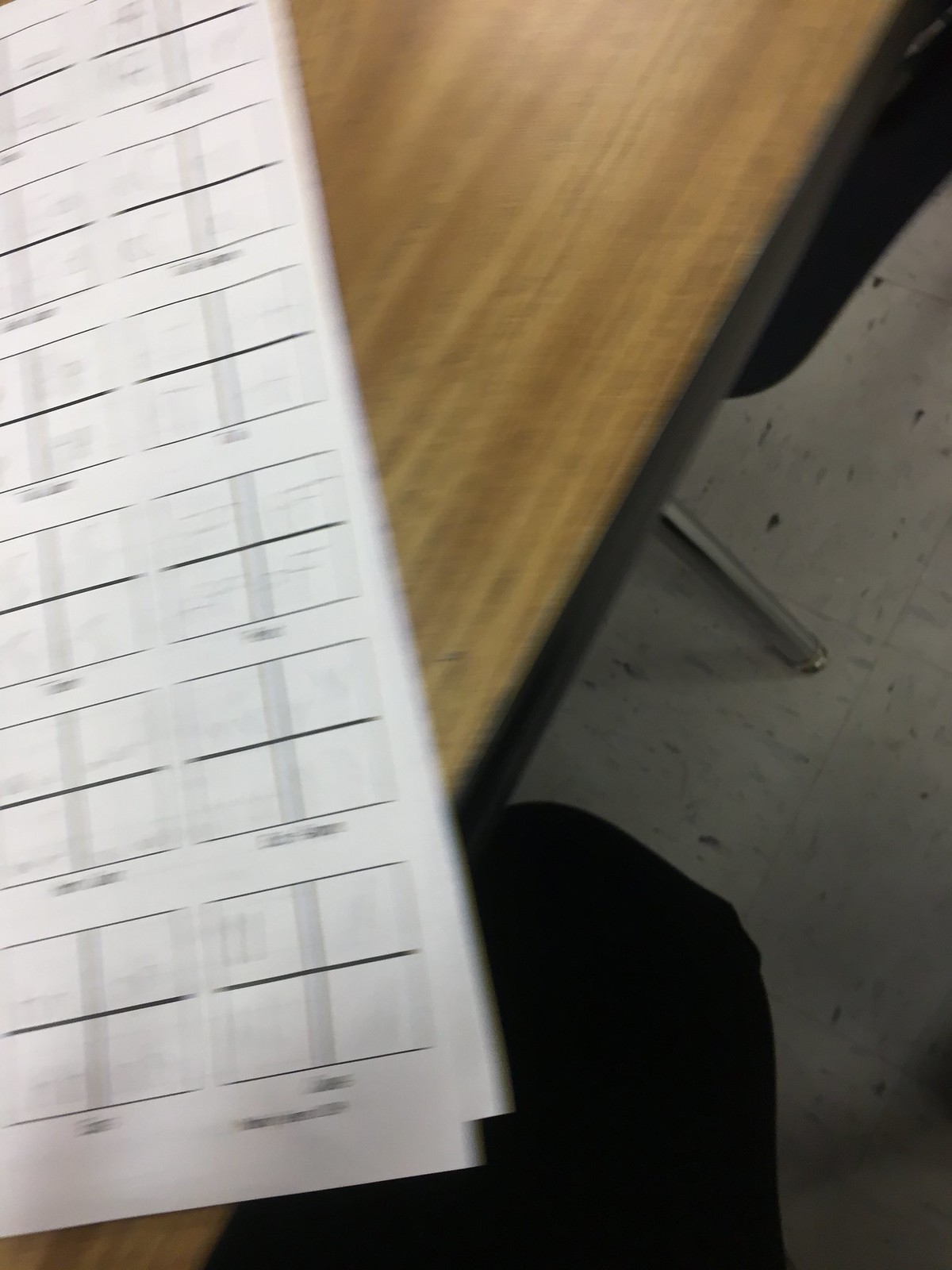This slightly out-of-focus photograph captures a person sitting at a table in an environment with light gray tiles reminiscent of school flooring. The table, featuring a plastic frame with metal legs, has a faux wood grain surface that gives the appearance of being wooden. Underneath the table, the person’s legs are visible, clad in black pants. On the table, there are two sheets of white paper positioned in front of the person. The top sheet displays a grid pattern with rows of square blocks. Each block is defined by a dark, thin line running horizontally from left to right and a thicker, lighter line running vertically from top to bottom.